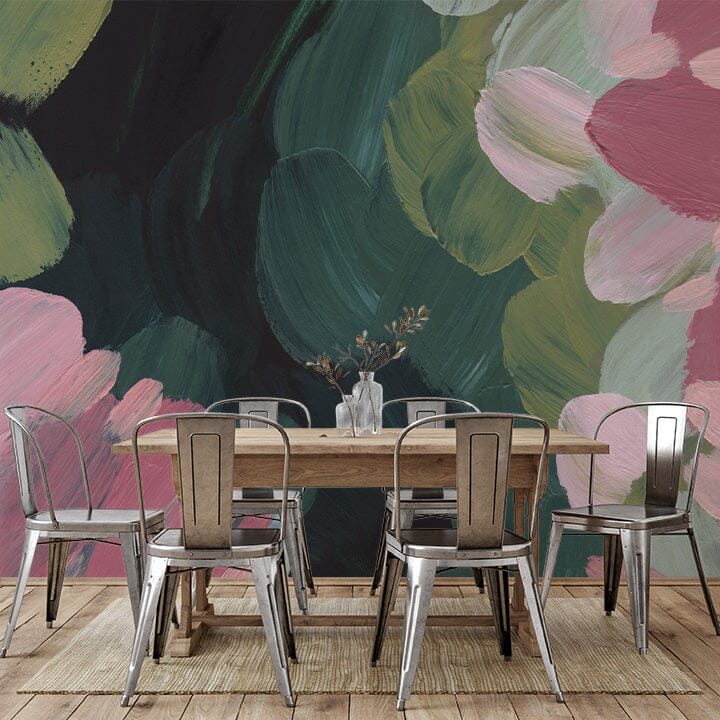This photograph depicts a simple yet elegant dining room or restaurant area with a striking blend of minimalism and artistic flair. The room features a brown, slatted wooden floor adorned with a blondish or natural wood mat, anchoring a prominent light wood grain table at its center. Surrounding the table are six stainless steel chairs, two on each of the longer sides and one at each end. Atop the table are two clear vases, each holding stems with brownish leaves. The background is dominated by a large, visually captivating mural, which uses an array of vibrant watercolor brushstrokes in shades of light green, dark green, pink, and rose, arranged to evoke a floral and petal-like aesthetic. This mural enhances the room's ambiance, providing a picturesque and serene backdrop to the simple, functional furnishings.